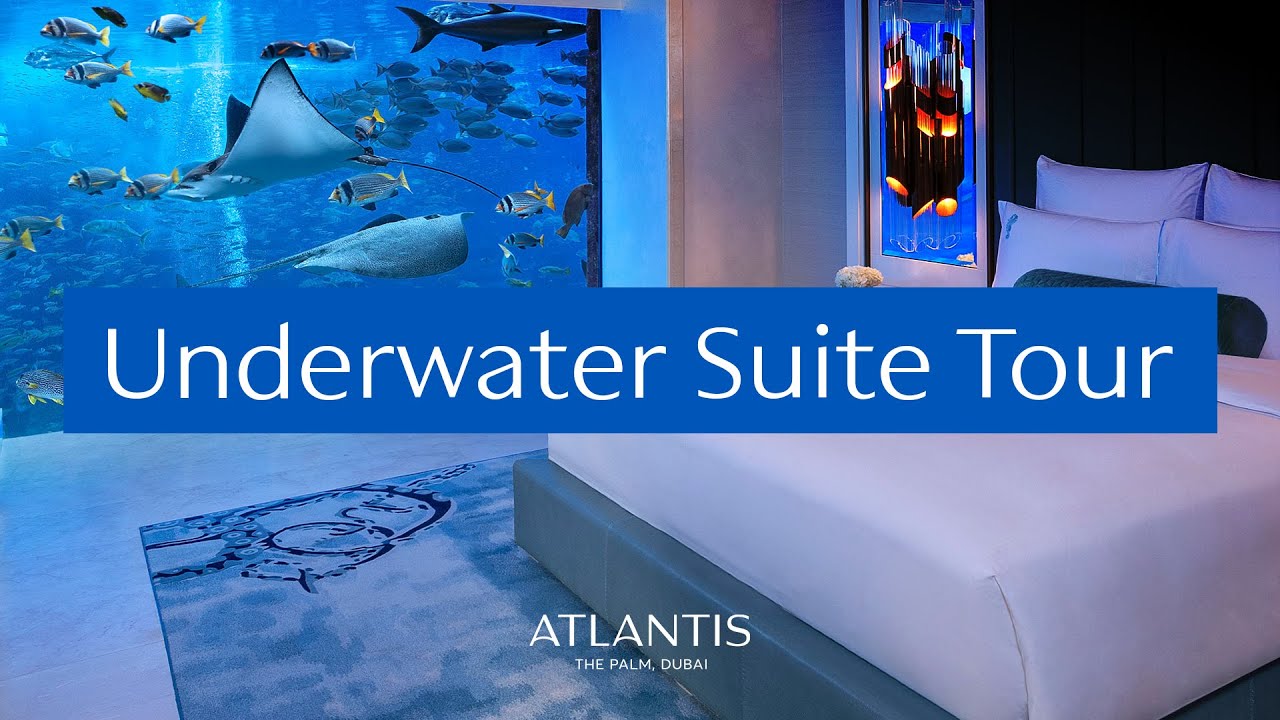The image appears to be an advertisement or flyer for an "Underwater Suite Tour" at Atlantis, The Palm Dubai. Dominating the scene is a hotel room with a bed featuring white bedding and pillows. Adjacent to the bed is a striking large aquarium wall teeming with an array of fish, including angelfish and sharks. A blue banner with white text reading "Underwater Suite Tour" spans the middle of the image, with "Atlantis, The Palm Dubai" written below it. Below the bed, there’s a blue and black patterned rug that contrasts the oceanic blue hue of the floor and the stunning blue waters of the aquarium. The room’s wall is white, accented by an abstract piece of artwork in black, orange, and blue, adding a touch of modern elegance to the aquatic theme.